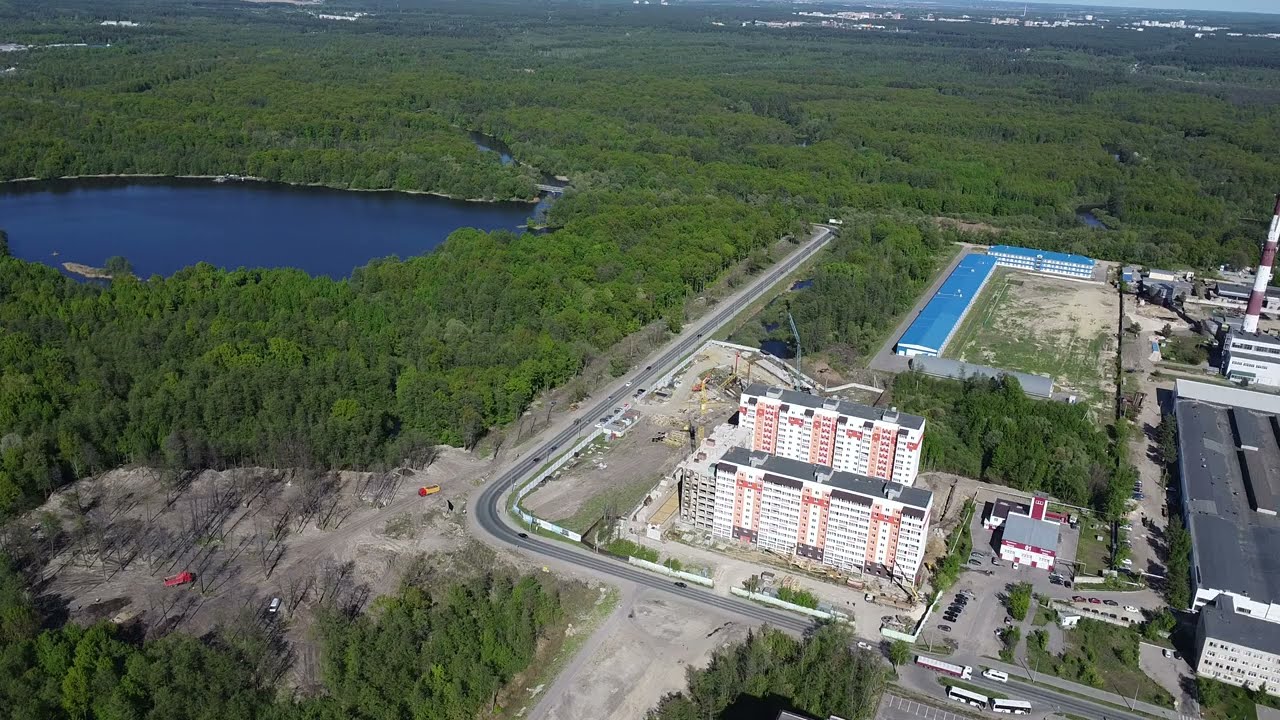This aerial view photo captures a sprawling, partially forested landscape intersected by winding roads and various buildings. Dominating the foreground, there is a large complex featuring a mix of tall and short buildings. Two of these buildings are particularly tall, with one reaching about 15 to 20 stories high and showcasing a striking white facade accented with red trim. Adjacent to this high-rise is a larger industrial building, approximately 4 to 5 stories tall, surrounded by smaller structures including a factory-like building with a blue roof and a prominent red and white smokestack.

Further into the distance, a lake glistens in the sunlight amid a sea of leafless trees, and beyond that, an expanse of forest stretches towards the horizon, giving way to some distant hilly terrain with scattered white patches. The left side of the image features a dirt clearing, indicating ongoing construction, where a red truck is visible. This area, devoid of trees, adds a contrasting texture to the otherwise green surroundings.

A rectangular framework of a two-lane road encloses the building complex, while an L-shaped road outlines the forested area. Various vehicles, including cars, trucks, and buses, travel these roads and are parked in a small lot between the large buildings. The bright, sunlit scene depicts a harmonious blend of natural and man-made elements, underscoring a landscape that is both industrially vibrant and densely wooded.